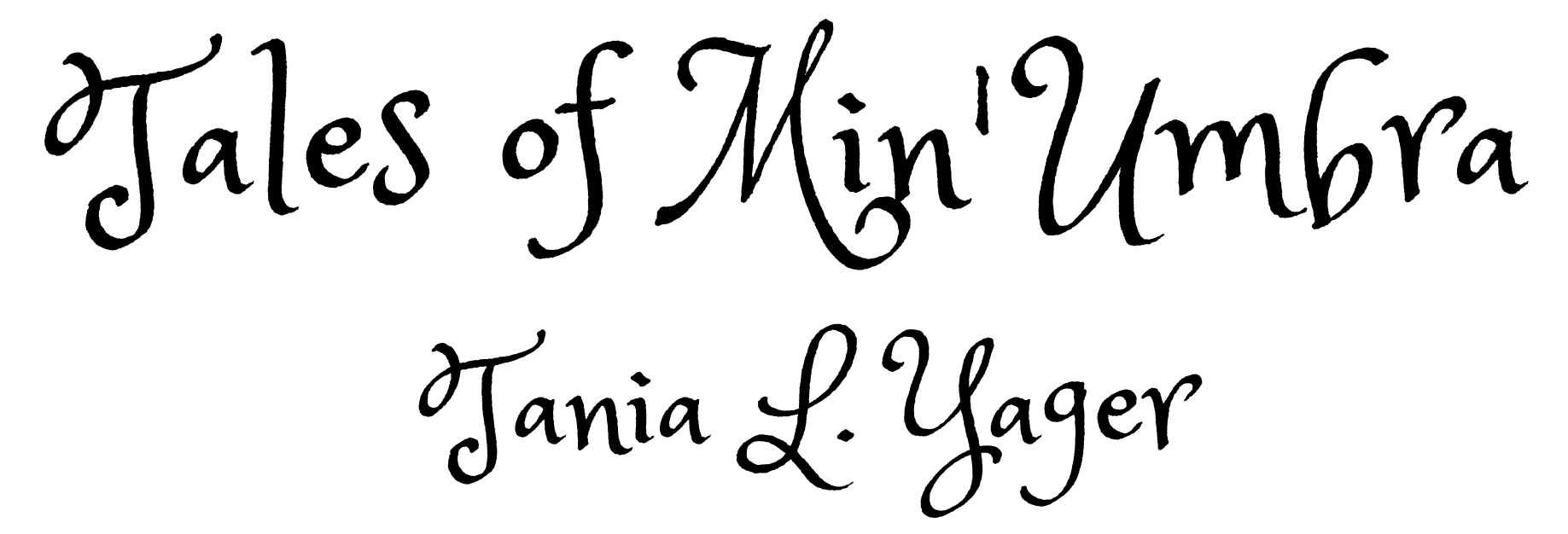This is a horizontal, text-based image with a completely white background that seamlessly blends into the page. The text, appearing in a whimsical handwritten script that resembles cursive writing with a black marker, reads "Tales of Min' Umbra" at the top. The font features ornate, swirly initial letters and an element of randomness, with characters slightly varying in height, contributing to a whimsical and uneven baseline. Below the title, in slightly smaller script, is the author's name, "Tanya L. Yeager," with each word beginning with a capital letter. The writing is bold and prominent, adding to the hand-drawn feel of the graphic.